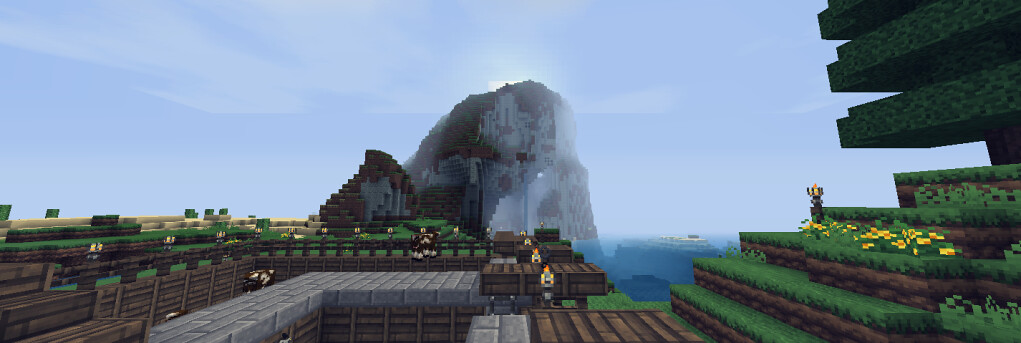Underneath a grayish blue sky, a majestic mountain stands at the center of the scene, its peak just beginning to catch the first golden rays of the sun. Wisps of clouds hover around the mountain, which appears to be constructed from large, block-like formations reminiscent of Minecraft, and features patches of brown amidst its predominantly gray surface. At the foot of the mountain stretches a vibrant green meadow, enclosed by a rustic wooden fence. The meadow is bustling with people walking from one end to the other, enjoying the serene landscape. To the right, a charming garden adds a splash of color with its grass-planted steps and clusters of bright yellow flowers, creating a picturesque and inviting atmosphere.